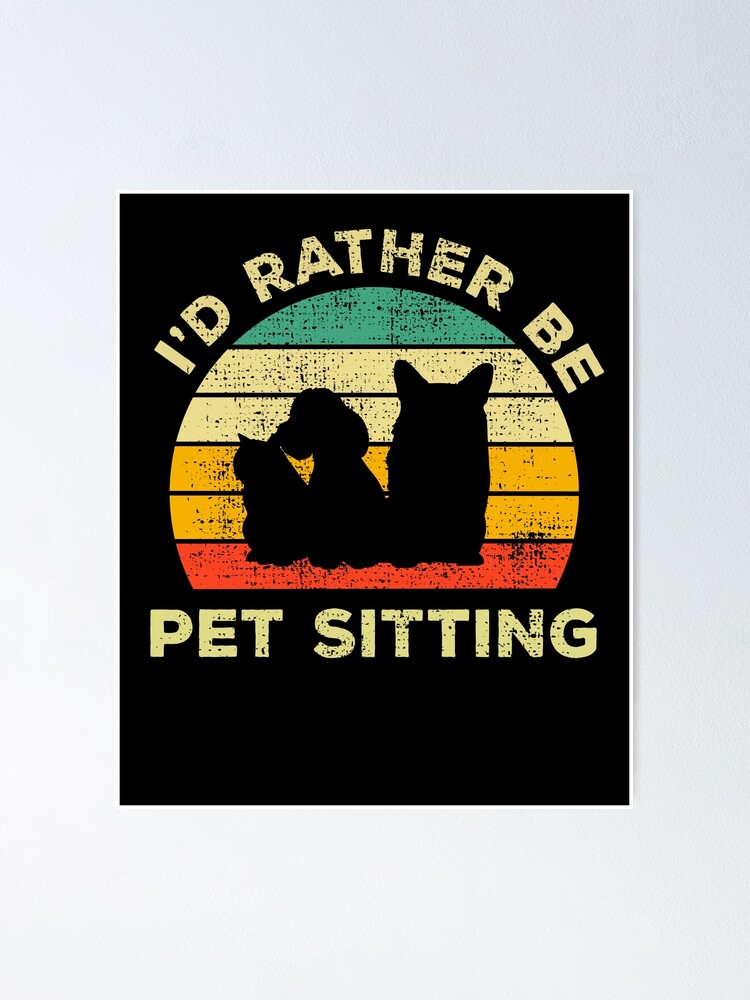This detailed caption integrates elements from all three descriptions, focusing on shared and repeated details:

"This image features a black sign with the statement 'I'D RATHER BE PET-SITTING' in bold, cream-colored capital letters. The sign, which could also be used as a bumper sticker or a decorative item in a home, car, or computer, showcases a vibrant design resembling a sunrise. The top semi-circle of the sunrise is filled with a gradient of colors including aqua, beige, yellow, orange, and red. The bottom part of the circle is missing, creating space for the text. The sign also features black silhouettes of three pets: a kitten, a beagle-like dog, and a small dog with erect ears. The entire image is set against a very light gray background, giving it a clean and modern look, and it may also serve as a design concept for a t-shirt."